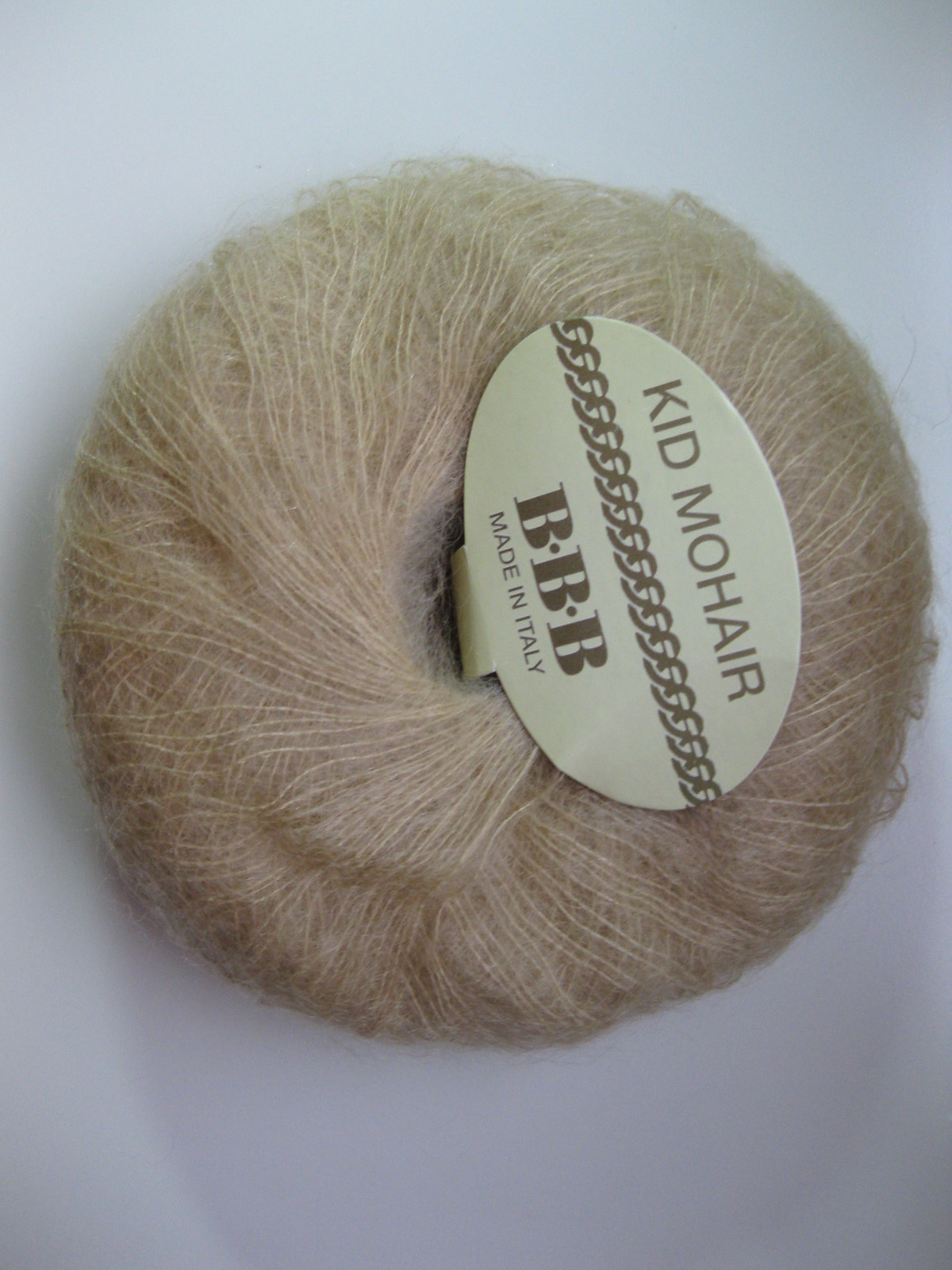The image features a close-up of a neatly wound ball of Kid Mohair, a type of wool, presented in a perfect spherical shape. The Kid Mohair is a sandy, blonde, or brownish-tan color with wider strands visible, giving it a textured appearance. It is set against a gray or beige background with varying shades, casting a shadow near the bottom of the image. A white cardboard label with a stitching-like graphic is prominently placed on the mohair. The label includes the text "Kid Mohair" in dark brown letters on a cream oval, along with "BBB" in capital letters, and "Made in Italy" written at the bottom. The arrangement suggests that this mohair ball is intended for crafts or fashion, possibly for spinning into yarn.